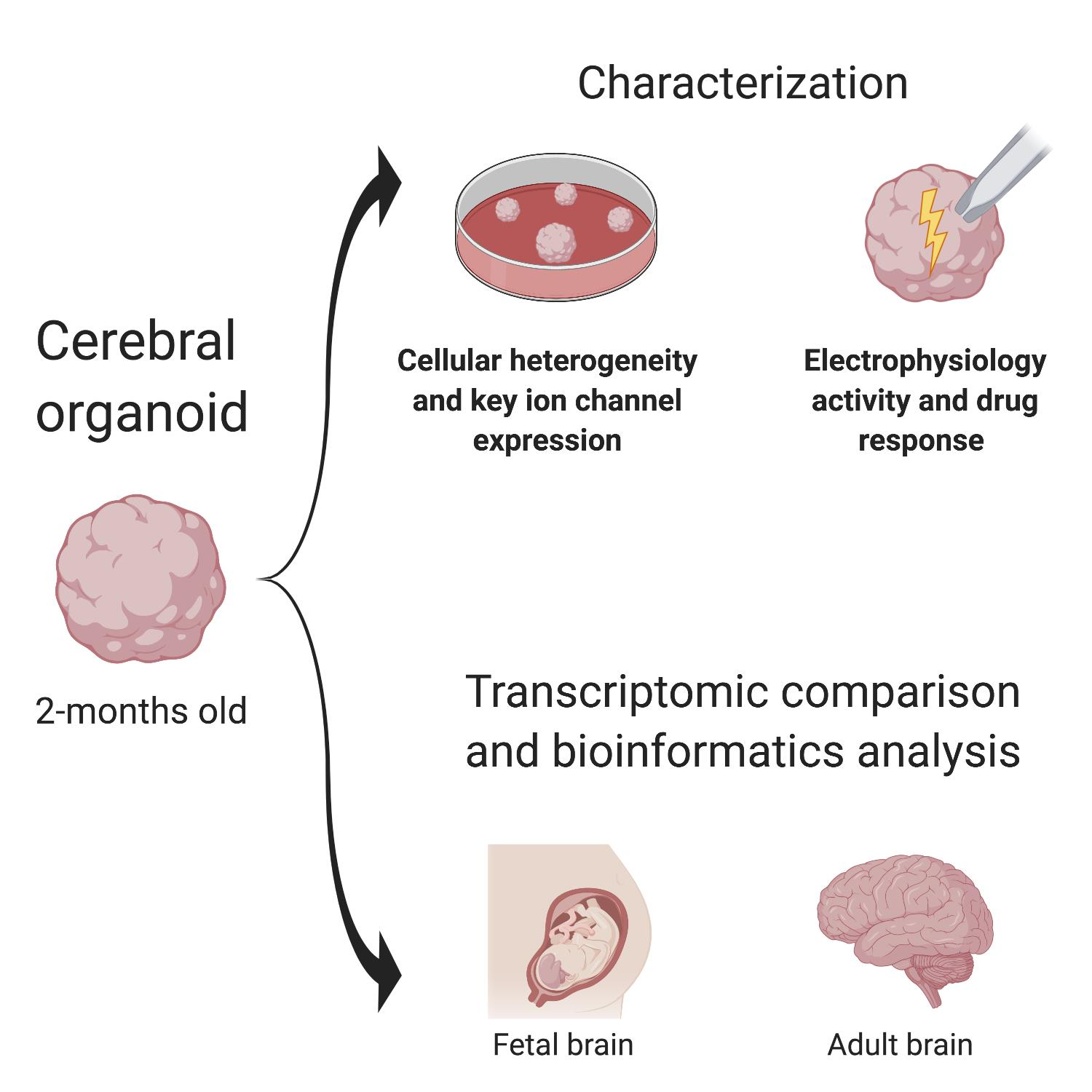The image is a detailed scientific flowchart, often found in textbooks or scientific journals, centered around the characterization of a two-month-old cerebral organoid, depicted as a pink, brain-like structure. The flowchart is titled "Characterization" at the top and begins with the cerebral organoid on the left side. Two arrows extend from this central organoid, one heading upwards and the other downwards, leading to different sections on the right.

The upward arrow points to a Petri dish labeled "Cellular Heterogeneity and Key Ion Channel Expression," alongside an adjacent image marked "Electrophysiology Activity and Drug Response," illustrated with a brain and a lightning bolt.

The downward arrow directs to the section labeled "Transcriptomic Comparison and Bioinformatics Analysis," which includes two subsequent images: one showing a fetal brain, visualized with a fetus inside a mother's womb, and the other depicting an adult brain. All brain-related depictions in the flowchart maintain a consistent pink hue.